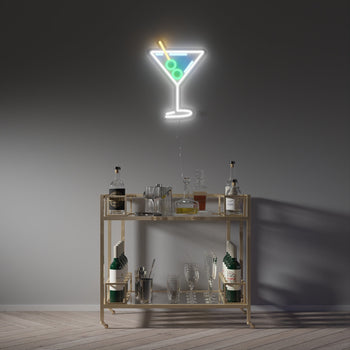The digital photo showcases a bar area within what seems to be a home, featuring a gray metal wine cart with two shelves. On the top shelf, there are several clear and possibly liquor-filled bottles, while the bottom shelf is lined up with four to five wine bottles, arranged single file on both sides. Between the bottles on the lower level, small spoons or stirrers and wine glasses are neatly placed. The wall behind the cart is a gradient gray, becoming lighter towards the bottom, and prominently displays a vibrant neon sign of a martini glass. The neon sign features two green olives with a stick and is illuminated with a combination of blue and white lights. The overall look of the space is minimalistic, with the distinctive neon sign adding a pop of color and character to the otherwise plain gray surroundings. The floor appears to be a grayish-brown, complementing the wall and the metal cart. Shadows of the cart cast sharply to the right due to the light reflection.